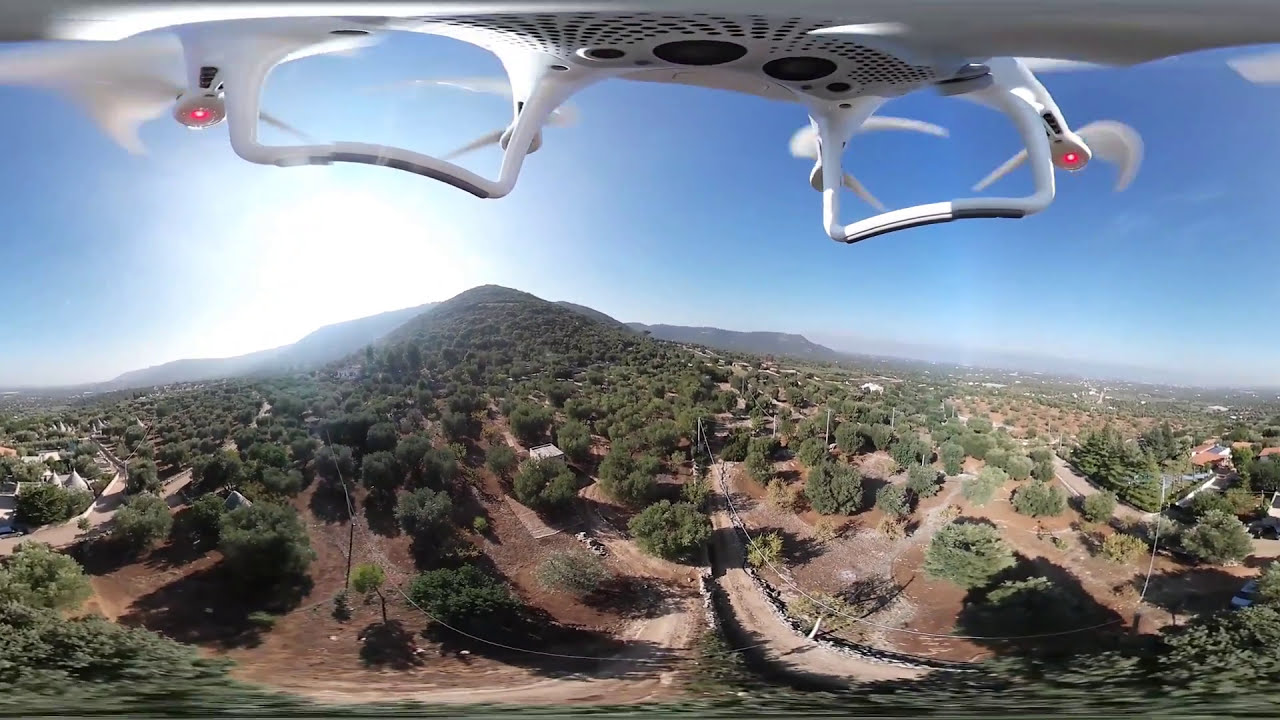This aerial image, captured by a drone, showcases a breathtaking landscape of rolling hills and a tall mountain range. The upper half of the photo includes the bottom portion of the white drone, complete with propellers and distinct red lights both at the front and back. The drone casts a shadow against a backdrop of green shrubbery and dense trees. The intricate terrain features a mix of greenery and earthy brown dirt areas, marked by a clearly visible dirt road bordered by electrical lines. The sky above is a bright blue, with the sun shining intensely from the left-hand side, illuminating the scene below. The image captures the serene beauty of the countryside with its green bushes and scattered buildings dotting the landscape, all under a clear, cloudless sky.